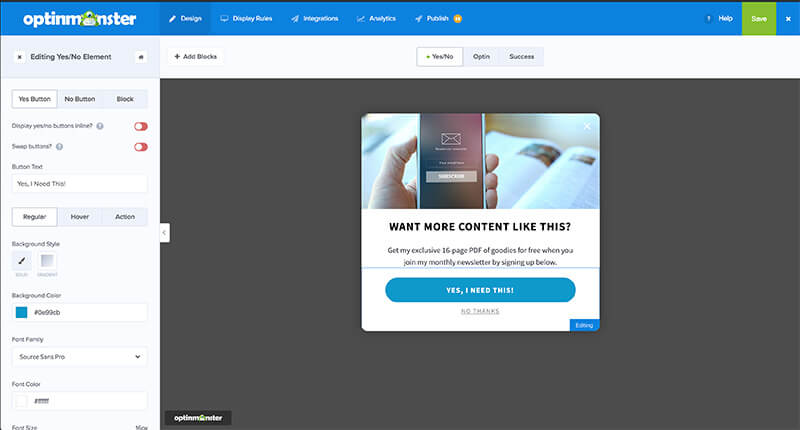This image is a detailed screenshot from the OptinMonster website, highlighting its design interface. At the top left corner, the website's name and logo—a green monster integrated into the "O" of OptinMonster—are displayed. The top section features a blue menu bar with various navigation tabs, including "Design," "Display Rules," "Analytics," "Publish," and "Integration." The "Design" tab is highlighted in a darker blue, indicating the current page. On the right side of this menu bar, there are icons for help (a question mark), saving changes (a green highlighted square), and exiting the website or tab (an X).

Beneath this primary navigation, the left sidebar on the design page presents multiple customization options. These include a section titled "Editing Yes/No Element" followed by three buttons labeled "Yes Button," "No Button," and "Block." There is also smaller text, albeit blurry, that seems to mention "Display Yes/No Button Inside" and "Sweep Buttons." Further options allow users to modify button text with settings for "Regular," "Hover," and "Action" states. Additional settings for background style, background color, font color, and font type ("Font Fancy") are also available.

The center of the page features a large, gray rectangle serving as the design area. Within this central design space, there is an example ad displaying a stock image of a person holding a phone. The ad message reads "Want more content like this?" Below the message, there is a prominent call-to-action button labeled "Yes, I need this," followed by a smaller, gray "No thanks" button. This screenshot gives a comprehensive view of the tools and options available for designing pop-up elements on the OptinMonster platform.